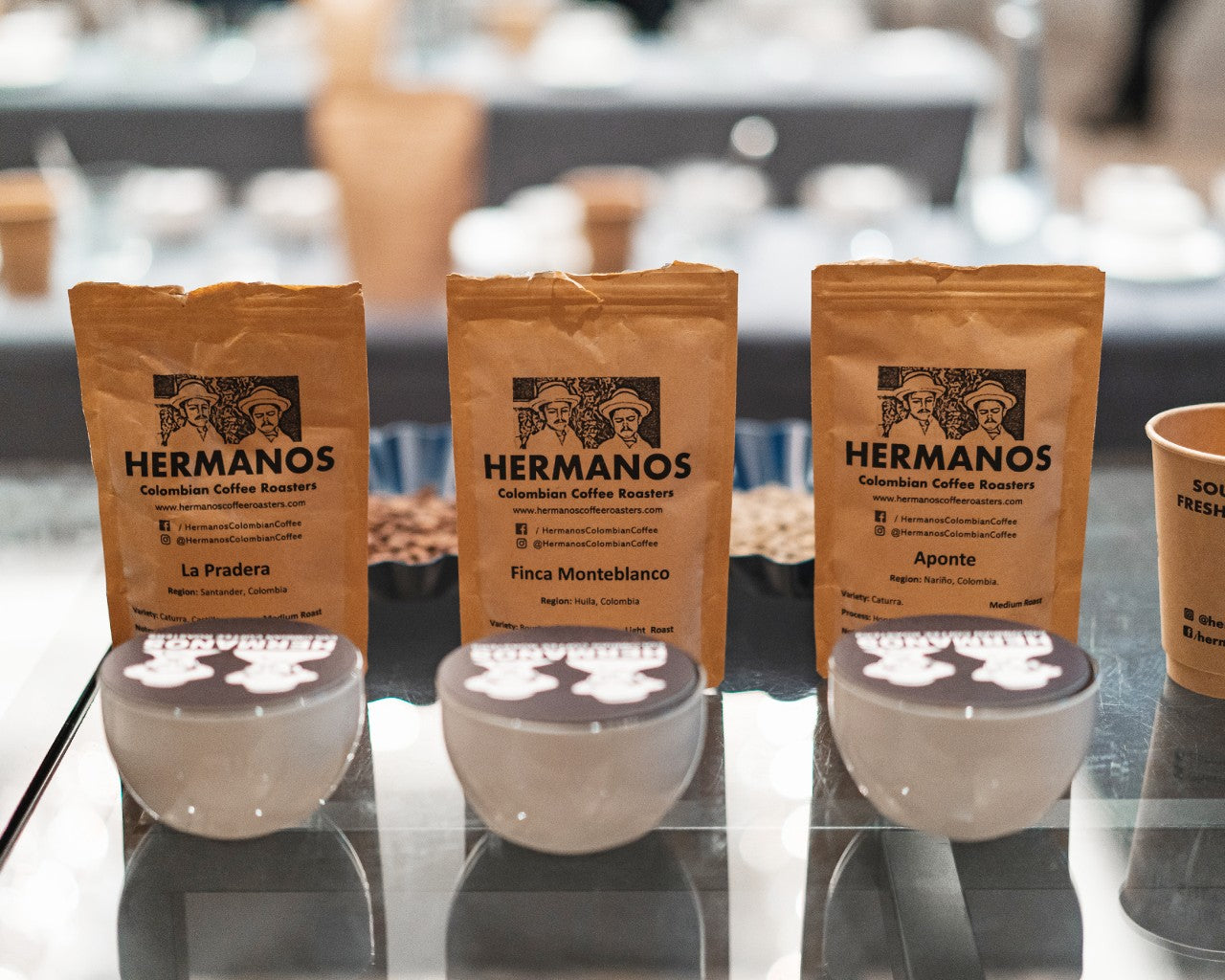In the foreground, a glossy gray table, divided into sections, showcases an organized display of Hermanos-brand Colombian coffee roasters. Prominently featured are three small, capped bowls, each emblazoned with the Hermanos logo, depicting a white outline of two men. Directly behind these bowls, three upright packets stand in a row, each package in vibrant orange and black, bearing the same logo and depicting the two men in a pencil-drawing style. The packets, with the variations La Pradera, Vinca Montablanco, and Aponte, highlight the different coffee flavors offered by the brand. To the right of the packets sits a tan coffee cup. In the blurred background, two long tables, one covered with a gray tablecloth, possibly display additional products or dinner dishes. The entire scene suggests a crisp, clean, and sophisticated presentation, focusing mainly on the Hermanos coffee products.